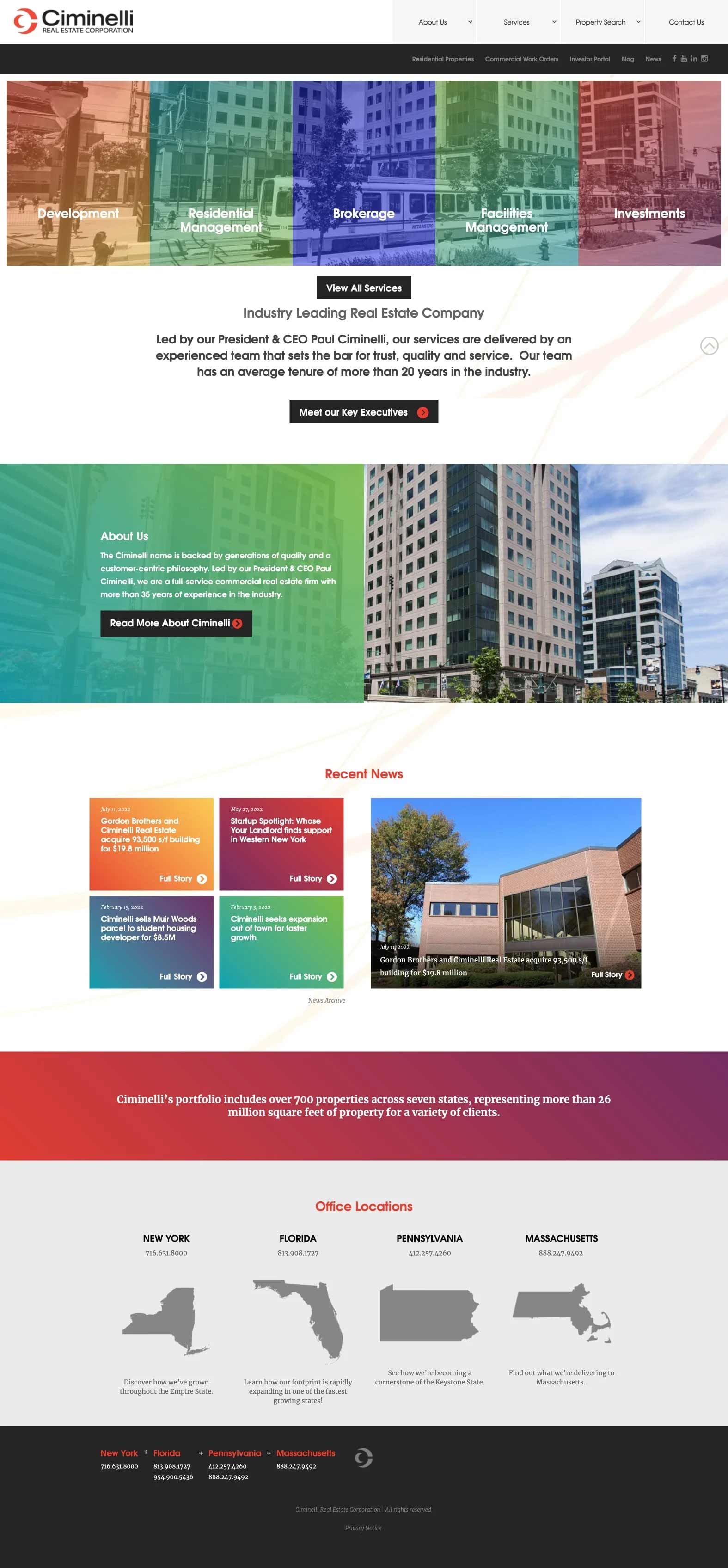The webpage for Ciminelli Real Estate Corporation features an organized and detailed layout. In the upper left corner, the company name "Ciminelli Real Estate Corporation" is prominently displayed. On the right side of the header, there are menu options aligned horizontally, starting in the center: "About Us," "Services," "Property Search," and "Contact Us," each with a pull-down menu for further navigation.

Directly beneath the header is a black band that spans the width of the page. On its right side, there are links to "Residential Properties," "Commercial Work Orders," "Investor Portal," "Blog," "News," and social media icons for Facebook and Instagram, along with an additional icon that is not clearly visible.

Below this black band, the page displays five colorful boxes in a horizontal row, each featuring a photograph. These boxes are labeled: "Development," "Residential Management," "Brokerage," "Facility Management," and "Investment," all in white font. A black button with white text labeled "View All Services" is located beneath these boxes.

Further down, a section highlights the company’s status as an industry leader in real estate, led by President and CEO Paul Corneli. It emphasizes their exceptional team, which boasts an average industry tenure of over 20 years, known for setting high standards in trust, quality, and service. A black button with white text and a red circle with an arrow is available for users to "Meet Our Executives."

Towards the bottom of the page, another section reiterates the company's commitment to quality and customer-centric philosophy, underpinned by the Corneli family name, which is synonymous with generations of excellence in real estate.